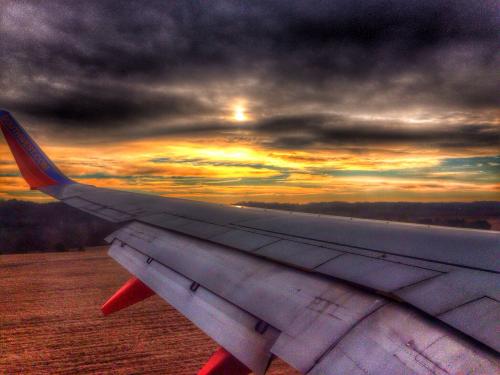In this evocative image, a silver airplane wing with distinctive blue and red tips extends from the bottom right corner to the middle left, set against a dramatic sky. The scene appears to be from a video game, capturing the wing from the perspective of a left-side passenger. Below the wing lies the ocean, while the background is dominated by a mesmerizing sky where the sun is either setting or rising. The sky boasts vibrant hues of yellow, orange, and red near the horizon, transitioning to darker shades of gray and black as stormy clouds gather above. The clouds themselves are thick and dark, hinting at imminent rain. Overall, the image is rich in color and detail, with the interplay of the bright horizon and the darkening sky creating a striking contrast.